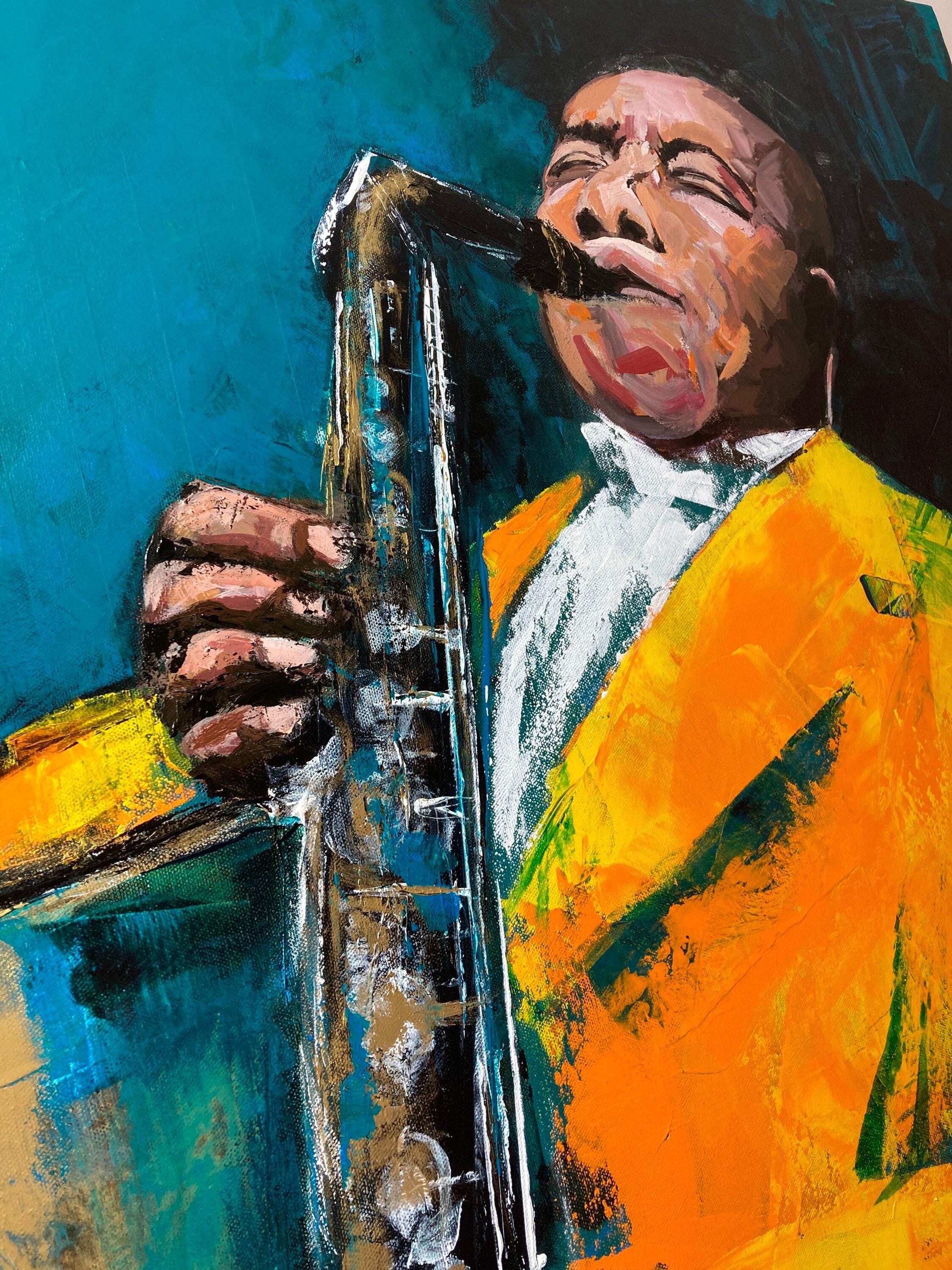This detailed artwork, rendered in chalk, depicts an African-American man playing a saxophone. He’s wearing a vibrant orange jacket with hints of green and a white shirt underneath. His eyes are closed, and his bald head tilts slightly as he immerses himself in the music. The saxophone, meticulously detailed with its keys and buttons, is positioned at the center of the image while the man stands slightly off to the right. The background features a gradient of teal to dark teal and black areas, enhancing the mood of the scene. One of the man's hands rests prominently on the saxophone, highlighting his engagement with the instrument. The overall composition evokes the soulful essence of a blues musician deep in performance.